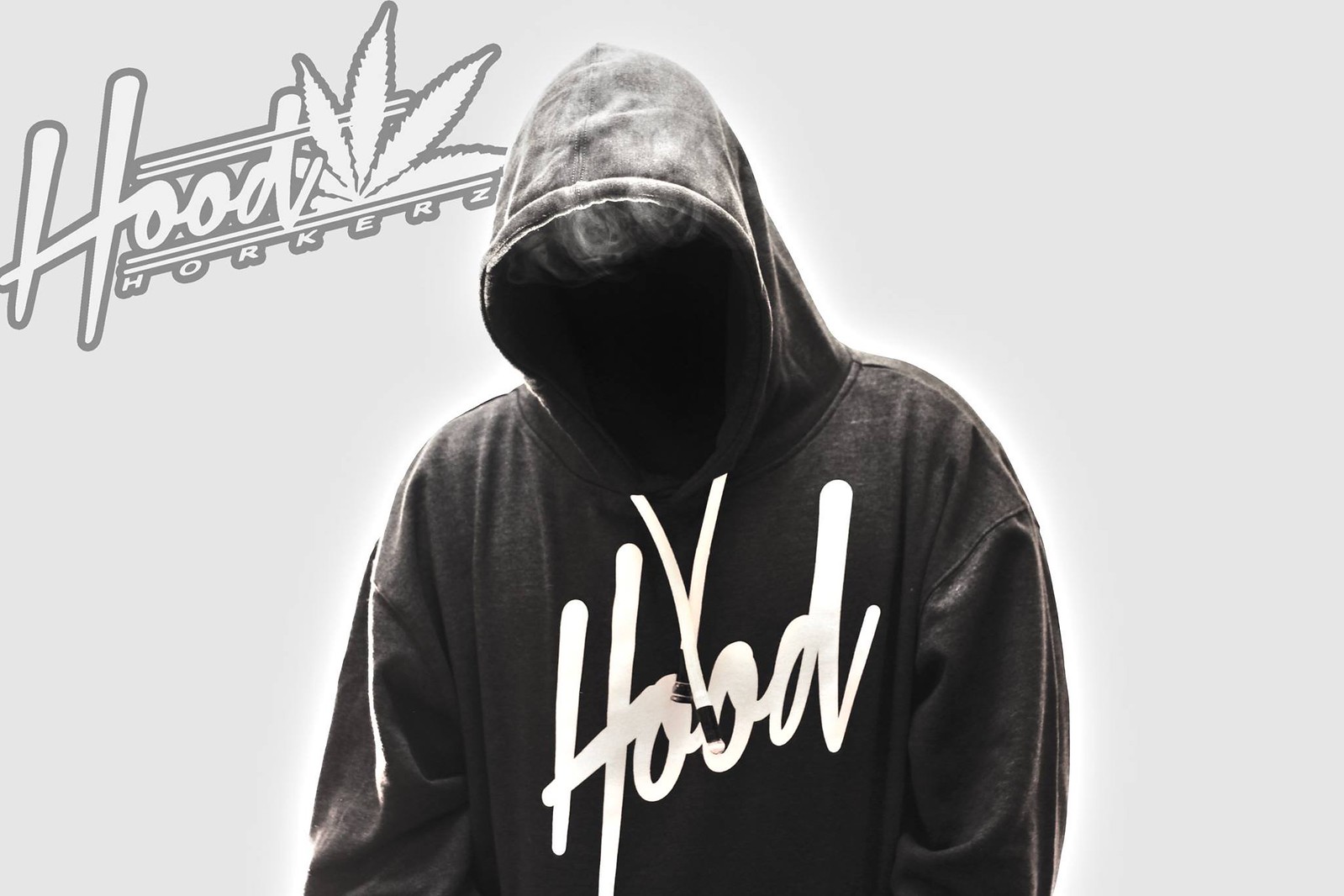The black-and-white advertisement features a striking, hooded figure set against a nondescript, light grey background. The individual, cloaked in a dark gray or black hoodie with bold, white cursive script spelling "hood" diagonally from the lower left to the upper right, remains mysterious, as their face is completely obscured. Billowing white smoke, likely from marijuana or a vape, emerges from beneath the hood, adding an enigmatic haze around the head. The hoodie also has two white drawstrings hanging down. The top left corner of the ad displays the brand name "Hood Horkers" in large, white letters with a light brown outline. Beneath this, a splay of marijuana leaves provides an edgy logo element. This eye-catching image, with its ghostly and rebellious vibe, subtly promotes the Hood Horkers brand while maintaining an air of cool anonymity.